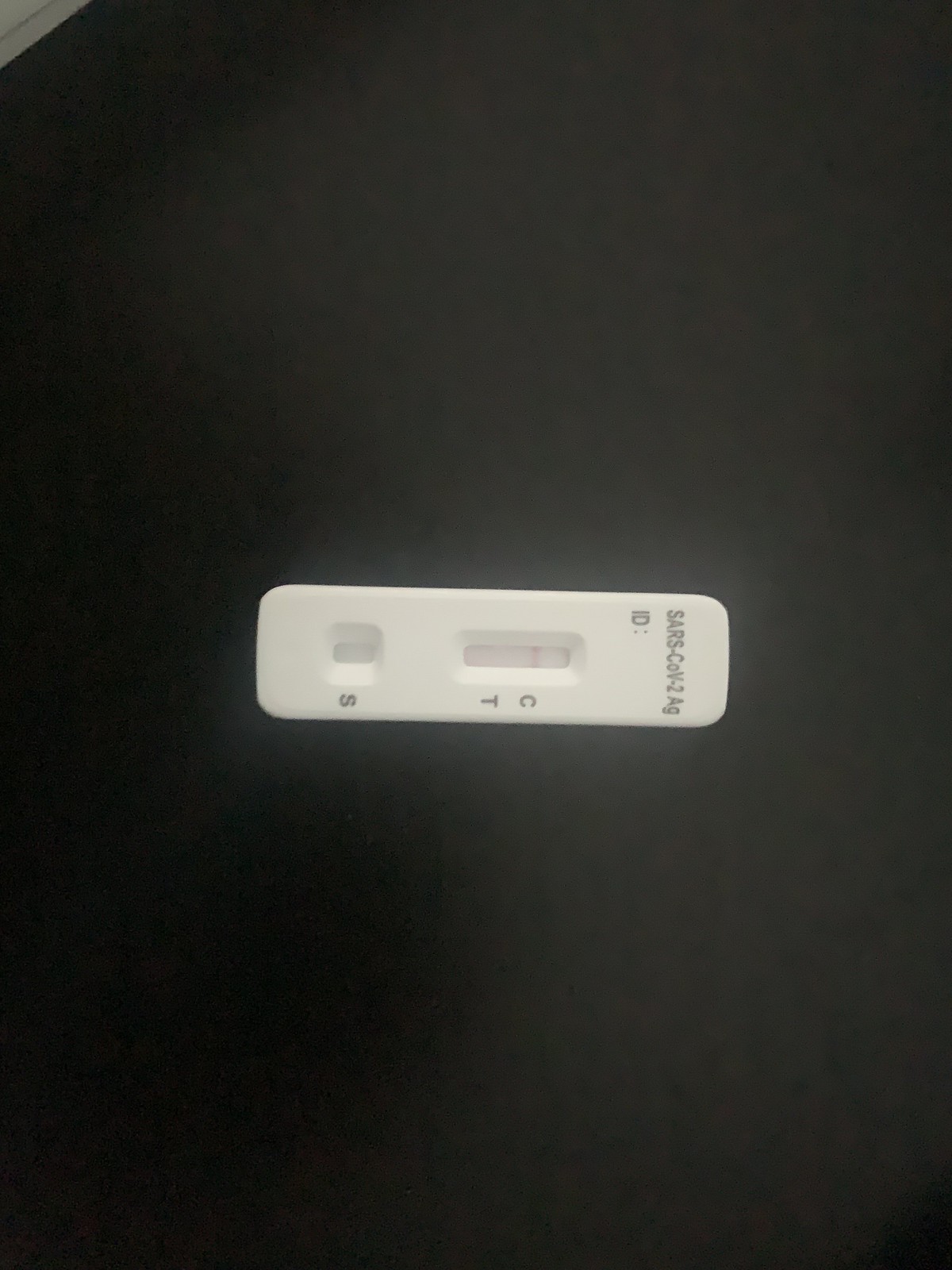The image portrays a COVID-19 testing device, viewed from a top-down angle. The testing device lies horizontally, with the label "SARS-COV-2 AG" prominently displayed at the top, followed by a blank field labeled "ID:". The device, resembling typical rapid test kits, is primarily white. It features designated areas marked with "C" and "T," as well as two grooved funnels. The "S" marking, next to one of the funnels, is the spot where the test sample is typically dropped. This sample is then guided into the upper chamber containing the "C" and "T" markers. 

Notably, a red line appears only next to the "C" marker, with no corresponding line next to the "T" marker, indicating a negative result for COVID-19. The top part of the device shows slight pinkish tones, hinting at where the test reaction occurs. The entire testing kit rests on a black table or bench, with a contrasting grey triangle visible in the top left-hand corner of the image, likely indicating the edge of a tablecloth or another surface transition.